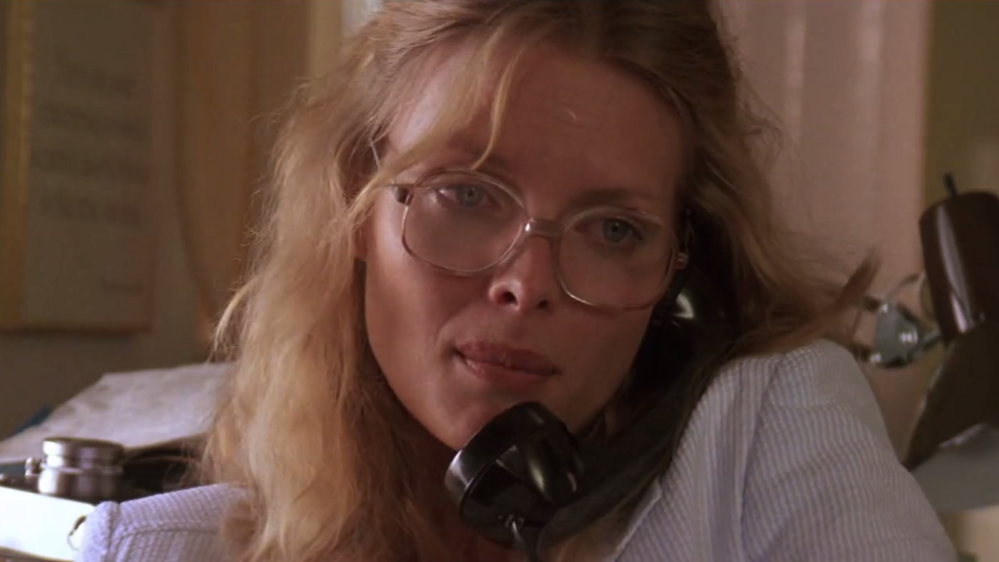In this wide rectangular image, we see actress Michelle Pfeiffer from a still that appears to be from a movie, likely taken sometime in the 80s or 90s. The top of her head is cut off, showing her from the shoulders up. Pfeiffer, with curly blonde hair that is somewhat wavy, tilts her head to the right diagonally while looking slightly down. She has large clear-lensed glasses and her lips are pink and pursed shut. She's holding a corded black phone to her left ear, suggesting she’s in the middle of a conversation. She is wearing a white shirt underneath a blue and white pinstripe blazer. The background features a mix of elements, including a gold or light pink colored curtain and a white wall with a framed picture that has some writing on it. There is also visible clutter behind her, adding to the room's somewhat disorganized appearance.